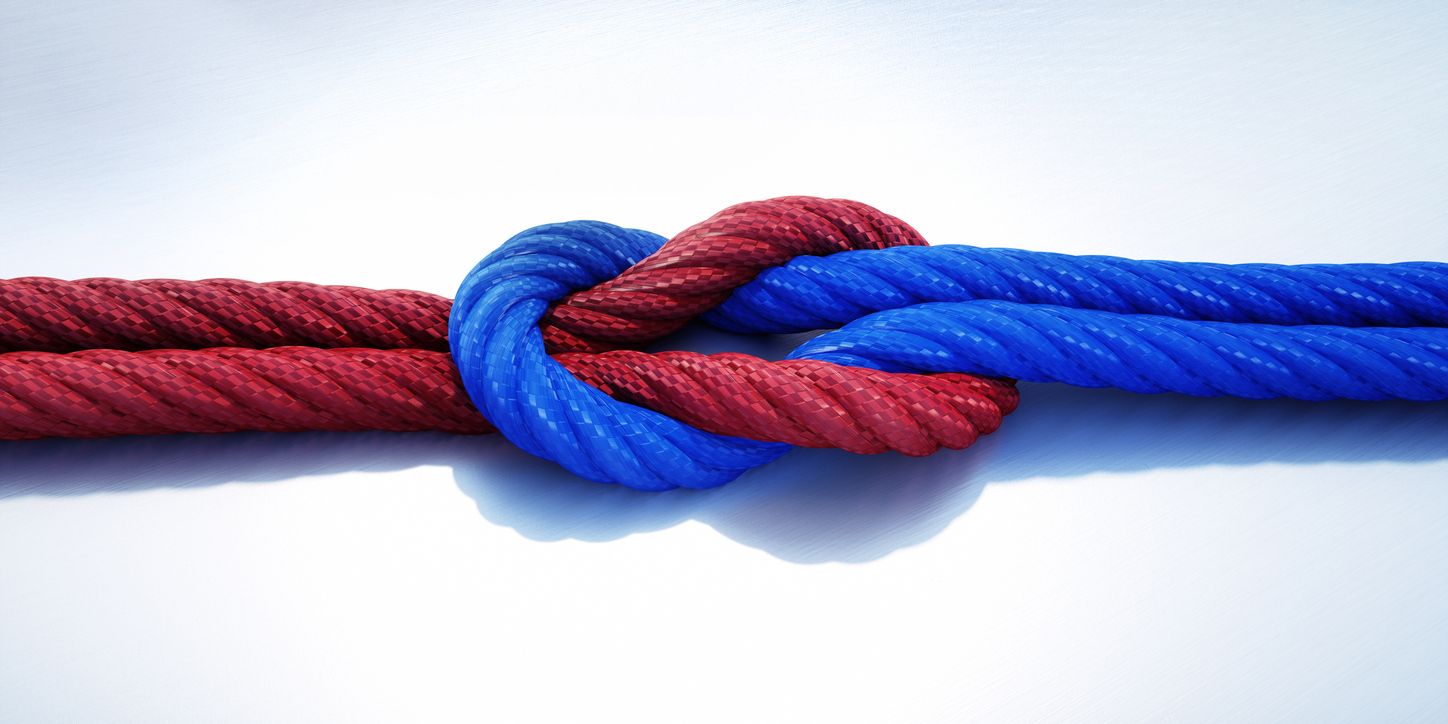The image features a hyper-realistic depiction of two thick ropes, one red and one blue, intertwined in a loose slipknot arrangement. The scene is set against a rectangular background that transitions from light gray at the edges to white in the center. The ropes, each approximately half an inch to three-quarters of an inch in diameter, create the illusion of two loops on the left side in red and on the right side in blue. These ropes interlock, with the blue rope's loops passing through the openings of the red rope and vice versa, forming an intricate, yet untightened, knot. The ropes stretch horizontally across the center of the image, casting subtle shadows on the white and gray background, suggesting a tangible, three-dimensional presence.